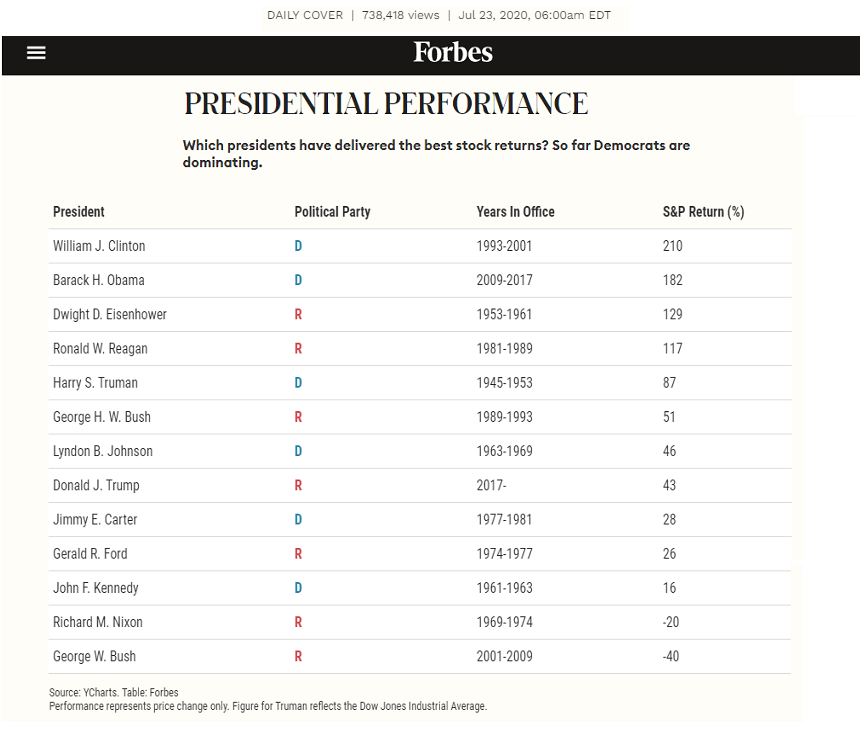This is a detailed chart from Forbes magazine, likely an excerpt from the July 23, 2020, issue and also available online, as indicated by an interactive menu button. The chart, titled "Presidential Performance: Which Presidents Have Delivered the Best Stock Market Returns?", provides a comprehensive analysis of stock market returns during the tenures of various U.S. presidents. The data includes the president's name, political party designation (D for Democrat, R for Republican), years in office, and S&P 500 returns in percentage. 

At the top of the list is Bill Clinton with a 210% S&P return, followed by Barack Obama, Dwight Eisenhower, Ronald Reagan, Harry Truman, George H.W. Bush, Lyndon Johnson, Donald Trump, Jimmy Carter, Gerald Ford, John F. Kennedy, Richard Nixon, and George W. Bush, who is at the bottom with a -40% return. Notably, the chart highlights that Democratic presidents, on average, have delivered better stock market returns. 

The colors representing political parties are the only hues visible on the otherwise white-faded graphic, which includes around 15 presidents, indicating its modern relevance with the inclusion of Donald Trump. The source is credited at the bottom as a "Why charts" table from Forbes, specifying that the performance represents price changes only and noting that the figure for Truman reflects the Dow Jones Industrial Average.